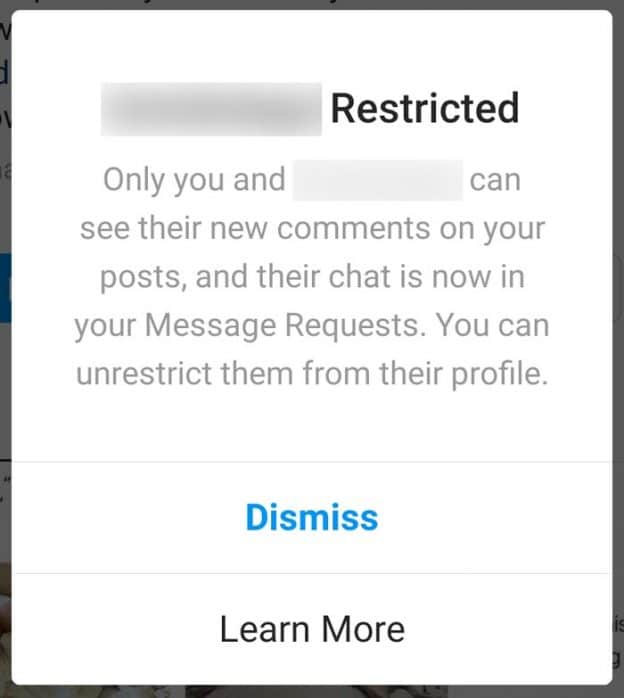A detailed descriptive caption for the image could be:

"This image captures a screenshot of a notification from a photo app, indicating that some words have been blocked out due to restriction settings. The notification primarily features the word 'restricted' prominently displayed at the top in bold black font, while the rest of the text is in gray. It informs the user that only you—and another obscured party—can see the new comments on your post. It also mentions that the conversation has moved to your message requests, and you have the option to unrestrict them from their profile. The interface provides two actionable options: 'dismiss' in blue and 'learn more.' The background is white and semi-transparent, partially revealing an obscured image of a person behind the pop-up notification."